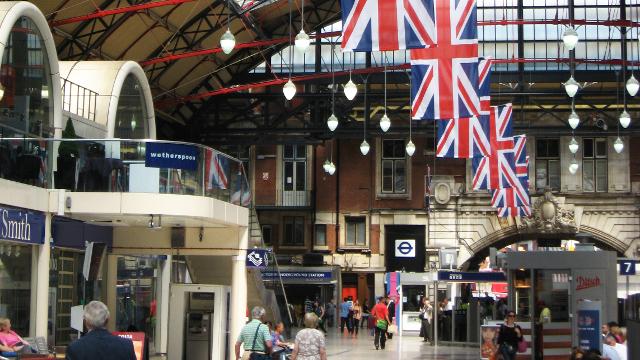This image captures the bustling interior of a large, old-style central train station, featuring a blend of modernity and vintage charm. The station's ceiling is tall, dome-like, adorned with metal rafters and beams. Hanging vertically down the center are rows of Union Jack flags, each suspended from red beam railings with pendant-style lights. The station boasts decorative stonework, notably around an archway, and appears to be a two-story structure with several kiosks and stands dotted throughout.

There is a prominent two-story store on the left-hand side, with a faded sign that partially reads "Weatherspoons" and another blue sign that says "Smith" in white letters. Shoppers bustle through the area, some passing by a small stand with a grayish front located towards the right, which appears to have a sign related to "Biscoff." The atmosphere is lively, filled with people seemingly oblivious to the photograph being taken, carrying on with their daily activities under the decorative flags and lights. The scene exudes a sense of timelessness, potentially suggesting the photograph dates back to the early 2000s or late 1990s.